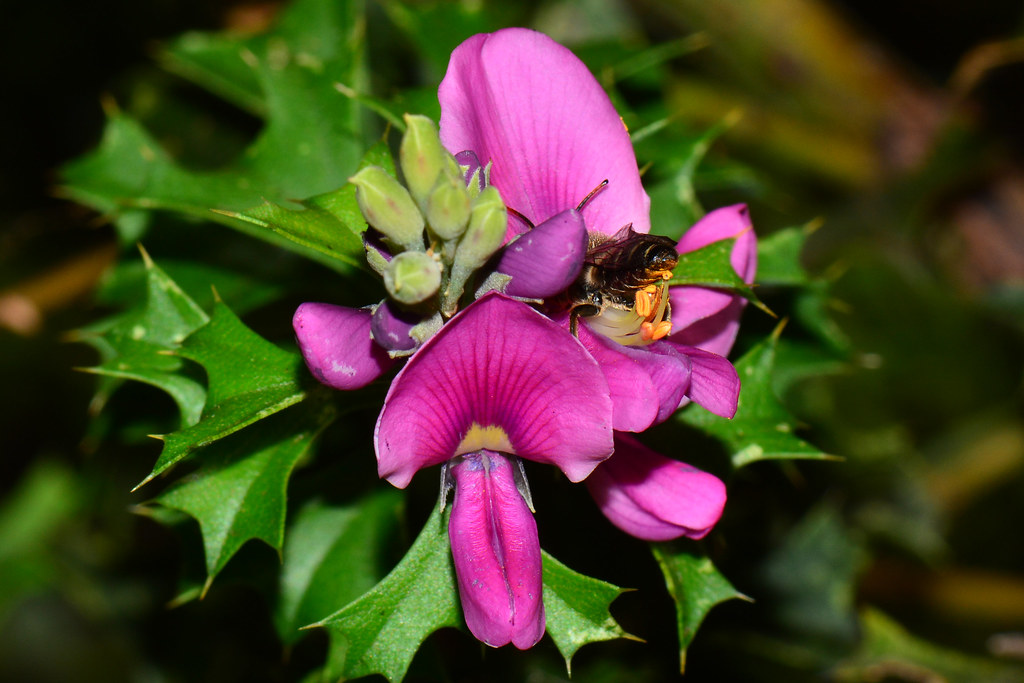This outdoor close-up photograph showcases a vibrant fuchsia, pinkish-purple hibiscus-like flower that evokes the floral beauty often associated with Hawaii. The main flower, which boasts an assortment of open petals and budding blooms, reveals hints of yellow at its very core. Prominently positioned in the center of the flower, a large bumblebee is busily collecting pollen, with its head immersed and back end, including its legs, distinctly visible. Surrounding the focal flower are glossy, bright green leaves with sharp, pointed edges that resemble thorns. The backdrop of the image is dark and blurred, featuring indistinct foliage that draws attention to the sharp clarity of the flower and bee in the foreground.